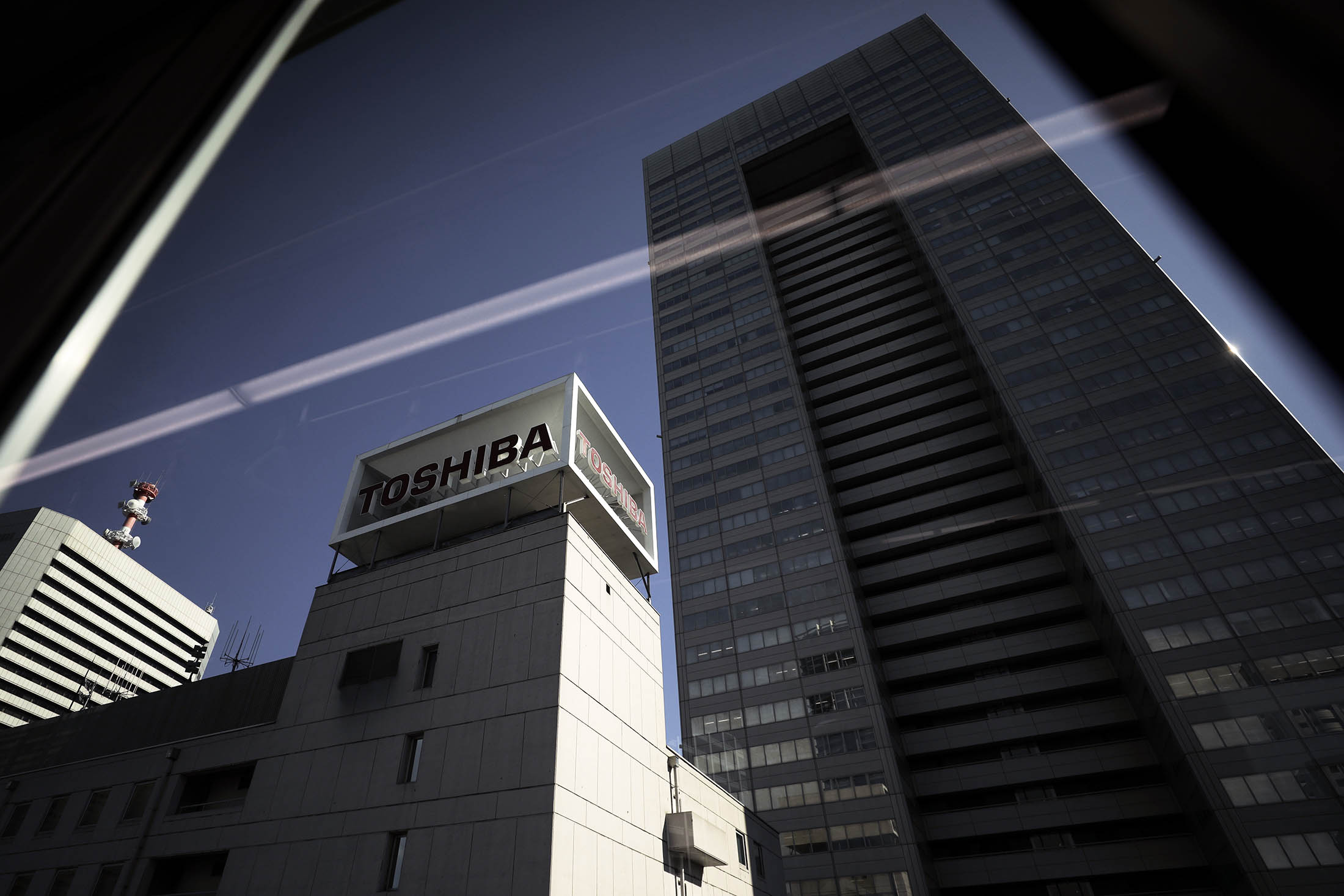This photograph captures a dramatic upward perspective of a modern city skyline, taken from the sidewalk looking vertically up at very tall skyscrapers. Central to the image is a striking gray and black skyscraper on the right, notable for its numerous horizontal lines and countless windows spread across at least 25 to 30 stories, creating an imposing and somewhat dreary presence. Adjacent to this behemoth, on the left side of the photograph, stands a building identified by the prominent "Toshiba" sign on its top two floors, suggesting it might be around five or six stories high but with only the uppermost levels visible in the image. Beyond these main structures, a third building's upper stories can also be seen peeking in the background. Adding to the complexity of the composition, a series of semi-transparent, diagonal white streaks—perhaps due to a glare or the reflection across a reflective surface such as a window—bisect the image, creating a triangular pattern and adding an additional layer of depth and intrigue to the upward view of the sky, which transitions from a light blue to a soft purple hue.